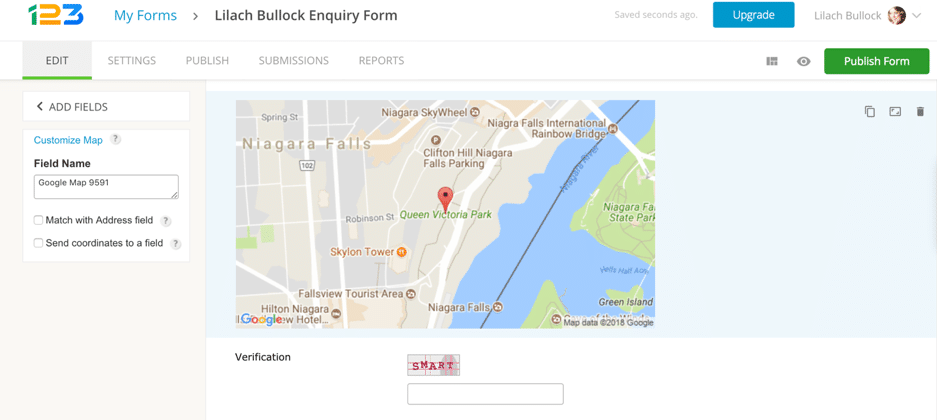The image is a screenshot from a website featuring a form editor interface. The upper left corner displays the website's logo, comprising a green '1', a yellow '2', and a blue '3'. Next to the logo, "My Forms" is written in blue text, followed by a right-pointing arrow icon. The main heading in black text reads "Lilach Bullock Inquiry Form," with "LiLACH" and "BULOCK" specified in more distinct lettering. To the right of this title, gray text indicates "saved seconds ago." There is a blue bar with "Upgrade" written in white text, followed by "Lilach Bullock" in gray text again, accompanied by a circular icon featuring a picture of a brown-haired woman.

Below this section, several tabs are visible: "Edit" in black with a green underline, "Settings," "Publish," "Submissions," and "Reports," appearing sequentially. To the right, a black box with an 'eye' icon is followed by a green click-able box with "Publish Form" written in white.

On the left-hand side of the main interface, there are two primary sections: "Add Fields" in black text, and "Customize Map" in blue text. Further down, there is a section labeled "Field Name," followed by "Google Map 9591" inside a white box. Subsequent options include "Match with Address Field" and "Send Coordinates to a Field."

To the right, a map showcases several landmarks around Niagara Falls. The upper left corner of the map pinpoints "Niagara Falls," accompanied by "Niagara SkyWheel" and "Niagara Falls International Rainbow Bridge." Blue water contours the map's depiction of Niagara Falls, with the name "Niagara Falls" marked near its bottom edge. Underneath the map, the word "Verification" appears in black text, while a red box labeled "SMART" and a blank box reside below it.